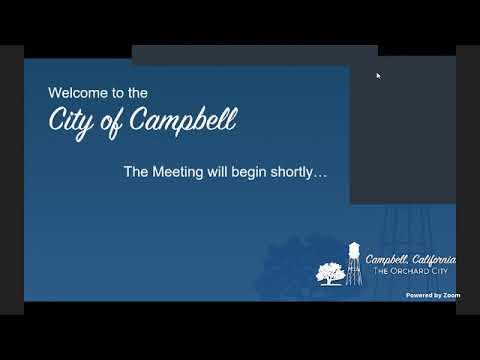The image is a screenshot from a Zoom meeting, potentially taken from a digital presentation or a TV screen. The layout features a black border with thin vertical dark gray stripes on the far left and right sides. The central area is dominated by a maritime blue rectangle, intersected by a gray rectangle on its right-hand side. In the top-left corner, white text reads, "Welcome to the," followed by a cursive script stating, "City of Campbell." Below this, centered, white text announces, "The meeting will begin shortly." In the bottom-right corner, white text specifies "Campbell, California, the Orchard City" alongside an illustration of a tree and a tall water tower. This illustration extends as a faint overlay on the maritime blue background. The lower-right corner also features the phrase, "powered by Zoom," in small white text.